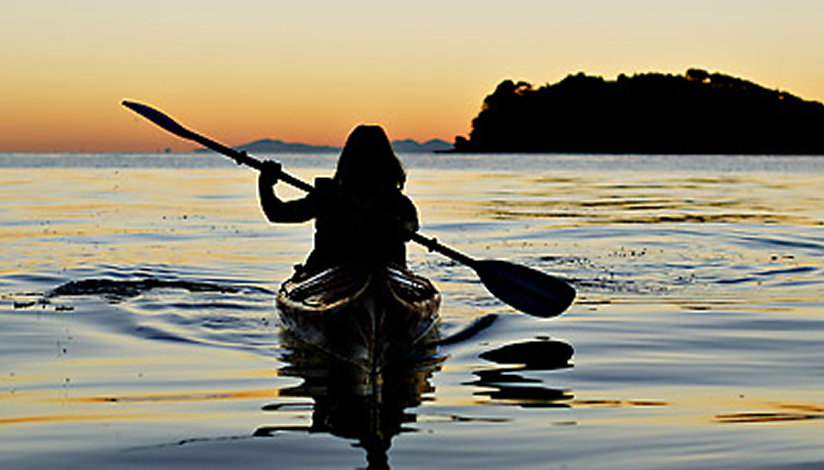In this evocative photograph, a silhouetted woman is pictured in a canoe, slightly off-center to the left, gliding gracefully over the water. Viewed from behind, her figure is cloaked in shadows, rendering her form entirely in black. Her shoulder-length hair catches the light just enough to outline its shape. The woman’s left arm is bent at the elbow, holding the top of an oar aloft with her hand, while the paddle's blade from the unseen right arm dips just above the water’s surface. The water itself presents a mesmerizing mix of deep blue and reflective yellow hues, hinting at the interplay of light and color. The sky above transitions dramatically from an unusual white at the top, down through shades of yellow and orange as it nears the horizon, creating a surreal backdrop. To the upper right, the dark silhouette of an island or a grove of trees adds a touch of mystery and balance to the composition.